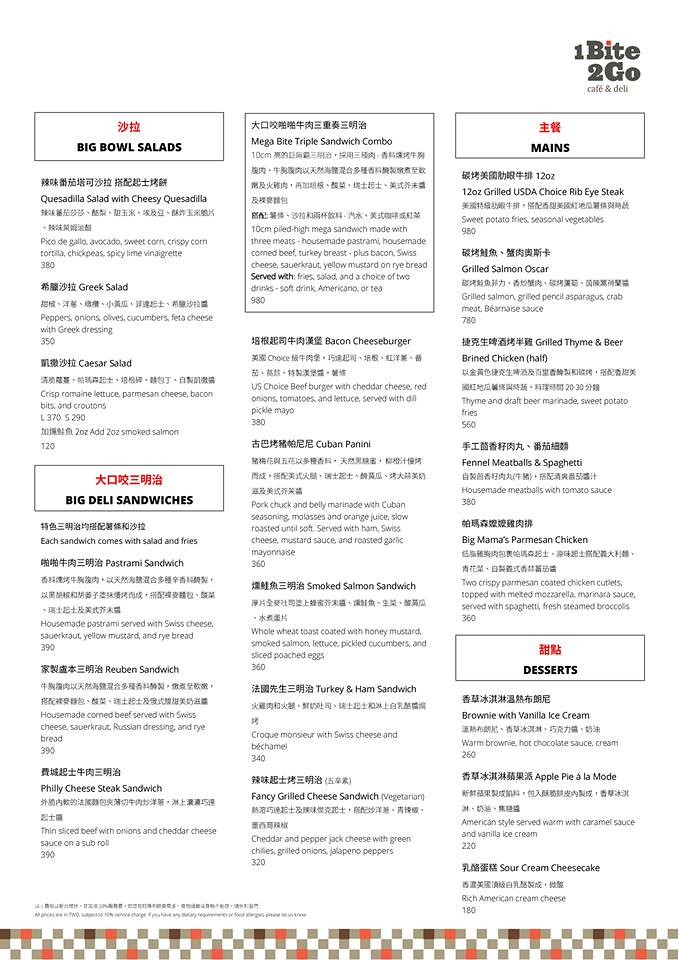The menu at the Chinese restaurant "One Bite Two Go Cafe and Deli" is divided into distinct sections, offering a wide variety of dishes to satisfy every palate. The "Big Bowl Salads" section includes options such as the Quesadilla Salad with cheesy quesadilla, a Greek Salad, and a Caesar Salad. Moving on to the "Big Deli Sandwiches," the selection features decadent choices like Pastrami Reuben, Philly Cheesesteak, Mega Bite Triple Sandwich Combo, Bacon Cheeseburger, Cuban Panini, Smoked Salmon Sandwich, Turkey and Ham Sandwich, and a Fancy Grilled Cheese Sandwich. 

For the "Mains," diners can indulge in a 12-ounce Grilled USDA Choice Rib Eye Steak, Grilled Salmon Oscar, Brined Chicken, Fennel Meatballs with Spaghetti, and Big Mama's Parmesan Chicken. To end on a sweet note, the "Desserts" section offers tempting treats such as Brownie with Vanilla Ice Cream, Apple Pie a la Mode, and Sour Cream Cheesecake.